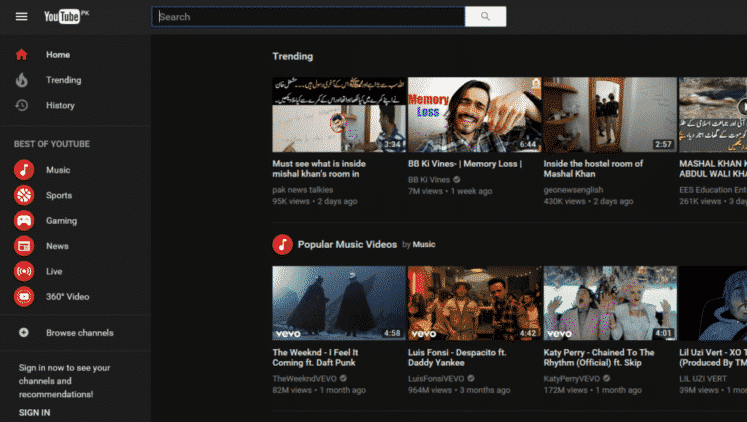The image depicts a dark-themed YouTube interface. On the left-hand side, a vertical menu lists several options, starting with a red icon labeled "Home." Below it are other sections: "Trending," "History," "Best of YouTube," with subsections for "Music," "Sports," "Gaming," "News," "Live," and "360 Video," all highlighted in red.

A notification prompt at the bottom of the menu reads, "Sign in now to see your channels and recommendations." The user is signed into the "Trending" section, where various video suggestions are displayed. The titles shown include: 

- "Must See What is Inside Michelle Kahn's Room"
- "B.B. King Vine's Memory Loss"
- "Inside the Hostel Room of Marshall Kahn"

Beneath the "Popular Music Videos" heading, several specific videos are listed:
- The Weeknd's "I Feel It Coming" featuring Daft Punk
- Luis Fonsi's "Despacito" featuring Daddy Yankee
- Katy Perry's "Chained to the Rhythm" (Official Video)

The overall aesthetic is dominated by dark tones, with highlighted elements in vivid red and white text.